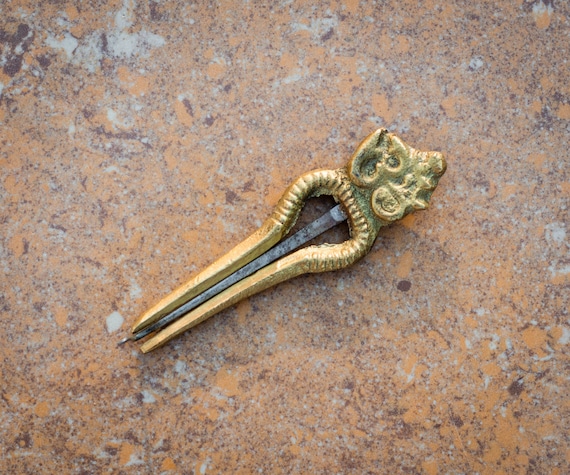The image depicts a detailed photograph of a vintage hair comb, possibly an ancient relic, made primarily of gold with intricate, ornate design. The comb features an animal head or face at the top, adding to its antique aesthetic. At its center, there's a silver or gray metal component, possibly acting as a needle or backplate that holds the hair in place. The object appears to be resting on a marbled or granite surface, characterized by a mix of tan, black, white, and orangey-red hues, suggesting it might be displayed for sale or as a collectible. The background’s marbled pattern with light orange and silver-black flecks accents the golden luster of the comb, making it the focal point of the photograph.